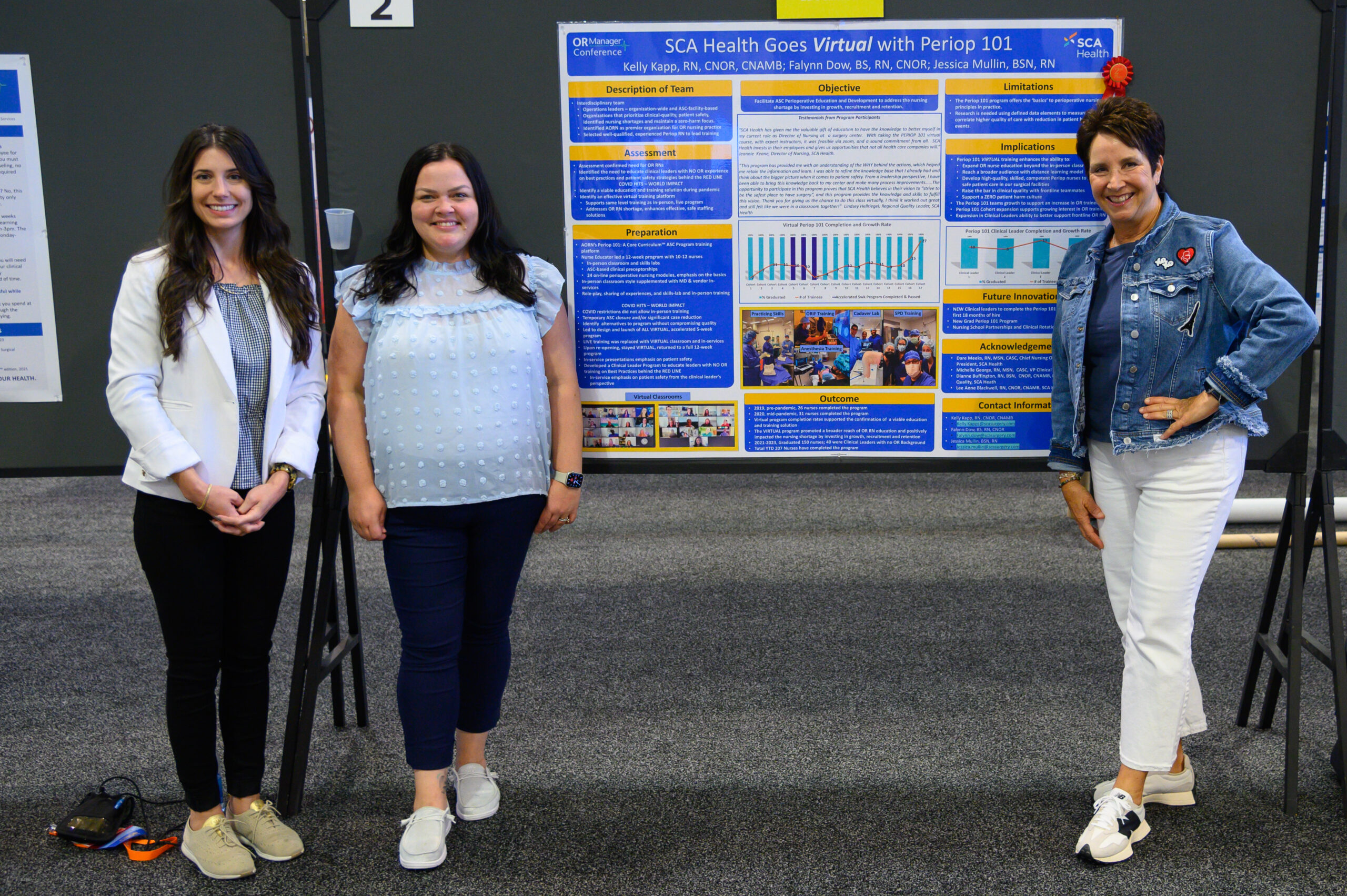The image features three dark-haired women standing in front of a prominent poster titled "SCA Health Goes Virtual with Peri-Op 101" at what appears to be a conference or exhibition. The poster includes detailed sections with headings such as description of the team, assessment, preparation, objectives, limitations, implications, future innovations, acknowledgments, and contact information, though the detailed text is too small to read. The board also lists the names Kelly Cap RN, CNOR, CNAMB; Phelan Dow BS, RN, CNOR; and Jessica Mullen BSN, RN. The background is gray, with a gray carpet underfoot, and there are additional exhibits slightly visible nearby, such as exhibit number two. The woman on the right, slightly older, wears a jean jacket, white pants, and poses with one hand on her hip. The woman in the middle has her arms at her sides, and the woman on the left, in her late 20s, stands with crossed hands at her waist. All three are smiling and dressed smartly, exuding a sense of pride and excitement. Electronics with visible plugs, possibly part of their demonstration, are seen on the floor to the left.